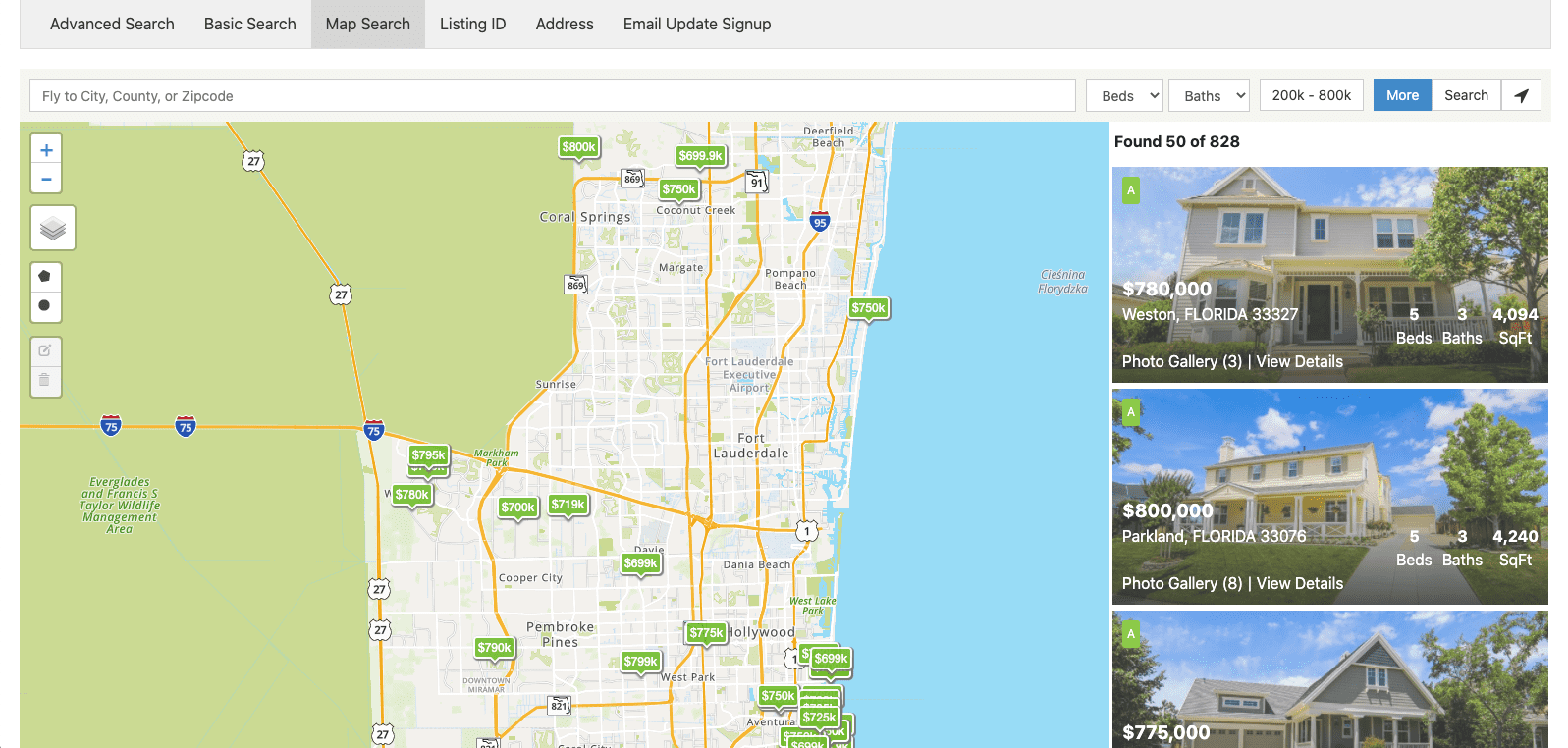A detailed screenshot of a property search interface displays a meticulously organized layout for house-hunting in Flattah City, Conway County, or specific zip codes. The top portion features a light gray background with a navigation bar in black lettering, containing options such as 'Advanced Search,' 'Basic Search,' and the highlighted 'Map Search' in darker gray. Additional options include 'Listing ID,' 'Address,' and 'Email Signup,' all surrounded by a subtle white border.

To the left, a prominent search bar guides users to enter their search criteria, flanked by dropdown menus for 'Beds' and 'Baths,' a budget range selector labeled '20K to 80K,' a blue 'More' button, and a white 'Search' button followed by an arrow pointing up to the right.

Below the search bar, the left segment of the screenshot portrays a light green map indicating regular land, transitioning to a white section intricately laced with orange street lines. Adjacent to the map's right side, a light blue body of water provides geographic context.

Prominently featured are three vertically stacked images of houses. The uppermost shows a grand two-story white house with a verdant tree on the right and clouds hovering above. A caption in black text reads "Found 50 of 828." The bottom left corner of each house's image displays its price, location, and the number of available photos. The right side details the number of bedrooms, baths, and total square footage.

Below, a similar two-story white house features an expansive sky, a driveway to the right, a tree, and lush grass in the foreground. The third image, slightly cropped at the bottom, depicts a gray house, completing the visual lineup of potential homes in the desired area.